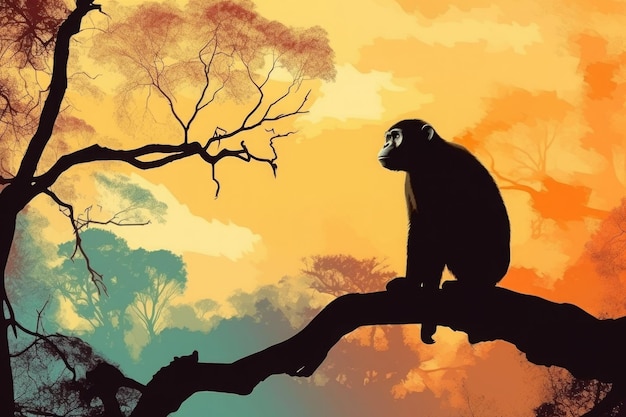This vivid digital illustration depicts a nearly silhouetted monkey perched on a black tree branch. The monkey, primarily rendered in black, has a white-highlighted ear and face, providing just enough detail to distinguish its features as it gazes off to the left. Surrounding the monkey are black branches adorned with maroon and bright red leaves. The background bursts with colorful tree silhouettes in diverse hues: a bright orange tree on the right, a muted mauve one in the center fading into a bright teal, all set against a sky painted in a radiant peach orange with lighter, almost white, orangey-peach clouds. The composition conveys a striking interplay of dark foreground elements and a richly colored, vibrant backdrop.